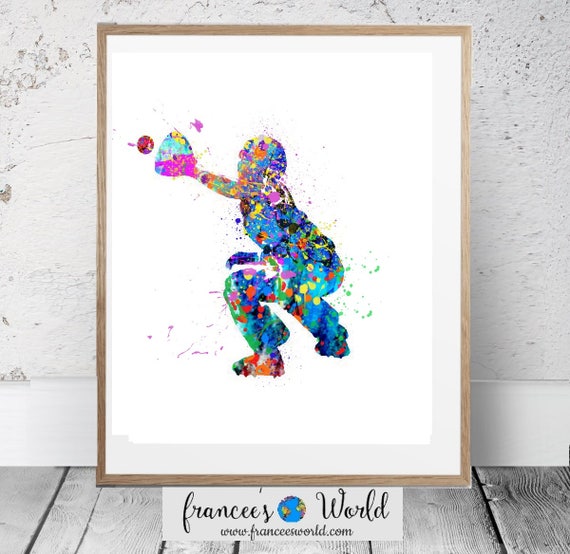The indoor image showcases a framed artwork piece, resting against a chipped white stucco wall, typical of a rustic, wooden-floored setting. The wooden frame encloses a psychedelic, multi-colored painting of a baseball catcher, crouched with an outstretched hand poised to catch a vivid red ball. The surreal figure, comprised of splotches in various hues including aqua, pink, and yellow, is clearly identifiable as a young boy playing baseball, though the abstract style gives it a tie-dye like appearance. The artwork is labeled with a graphic at the bottom that reads "Francis World" along with the URL www.francieworld.com.